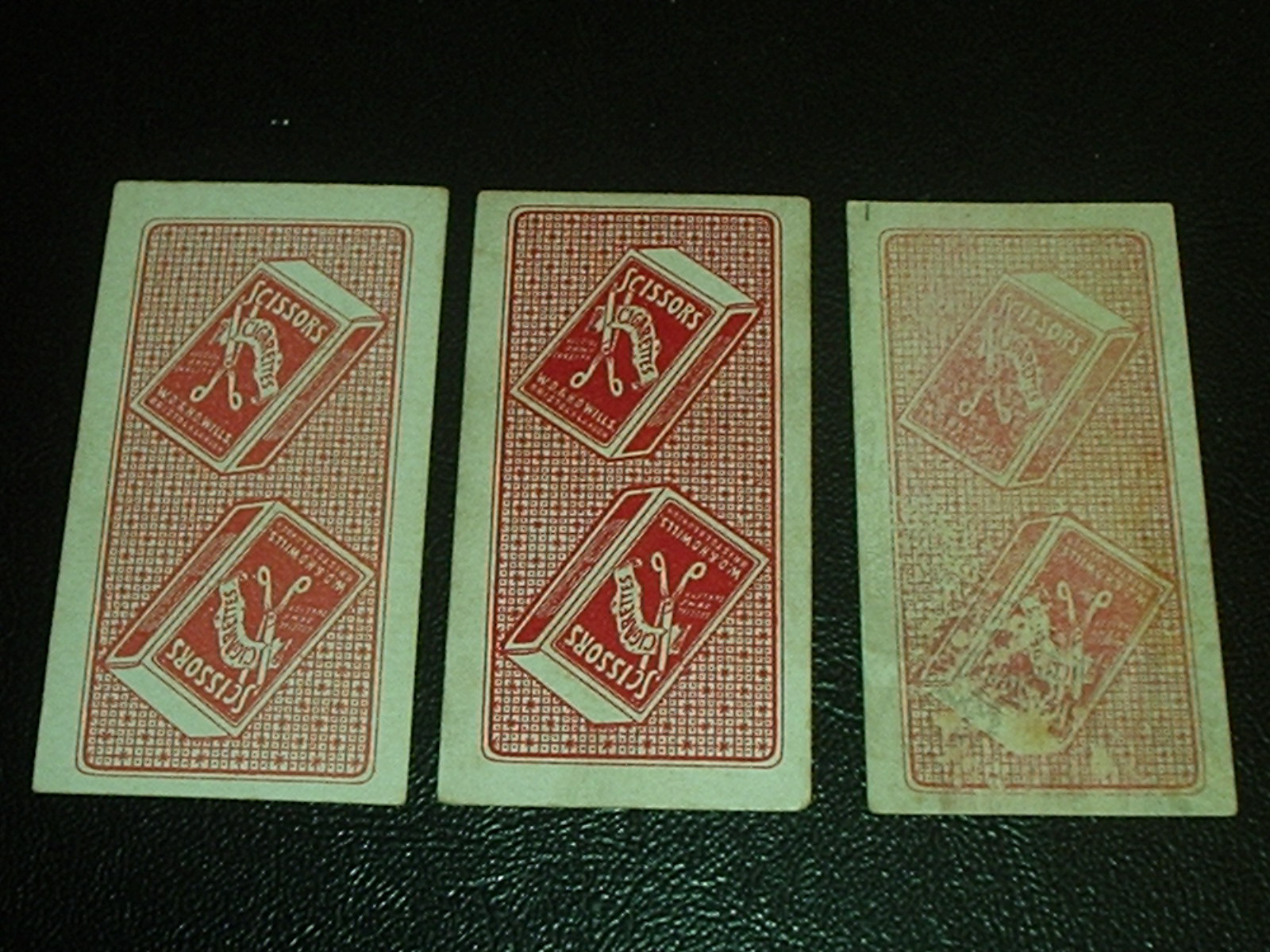This landscape-oriented photograph showcases three vintage advertising plaques, presumably from the 1910s to 1940s. These plaques, all made of the same cardstock, display varying degrees of preservation from left to right: medium grade, high grade, and very low grade. Each plaque features a red diamond pattern on white cardstock, with identical designs advertising Scissors Cigarettes. The leftmost plaque is in medium condition, displaying a moderately faded red hue. The central plaque is in excellent condition, boasting a vibrant, deep red color. Conversely, the rightmost plaque is significantly damaged, showing signs of water damage, dirt smears, and general wear and tear. All three plaques rest on a slightly textured, black vinyl-like surface, though the material is not definitively identifiable.